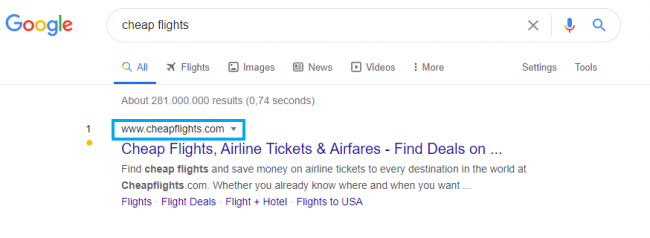The image appears to be a screenshot of a Google search results page with a clean, white background. In the upper left corner, the familiar Google logo is visible, showcasing its distinctive multi-colored letters: a blue capital "G," a red "o," a yellow "o," a blue lowercase "g," a green "l," and a red lowercase "e." 

To the right of the logo is a search bar where 'cheap flights' has been typed. Adjacent to the search bar, a microphone icon is present, indicating the option for voice search.

Below the search bar, several category tabs are visible, including "All," "Flights," "Images," "News," "Videos," and "More." The "All" tab is currently selected, signified by its darker shade. Further along the line, there are additional options titled "Settings" and "Tools."

The search results indicate approximately 281 million entries, retrieved in a swift 0.74 seconds. The first listed result shows the website "www.cheapflights.com," accompanied by a drop-down arrow, highlighted with a blue background.

The main title of this entry reads: "Cheap Flights, Airline Tickets, and Airfares - Find Deals On..." Below this, there's a brief description: "Find cheap flights and save money on airline tickets to every destination in the world at cheapflights.com. Whether you already know where and when you want...," followed by options for "Flights," "Flight Deals," "Flight + Hotel," and "Flights to the USA."